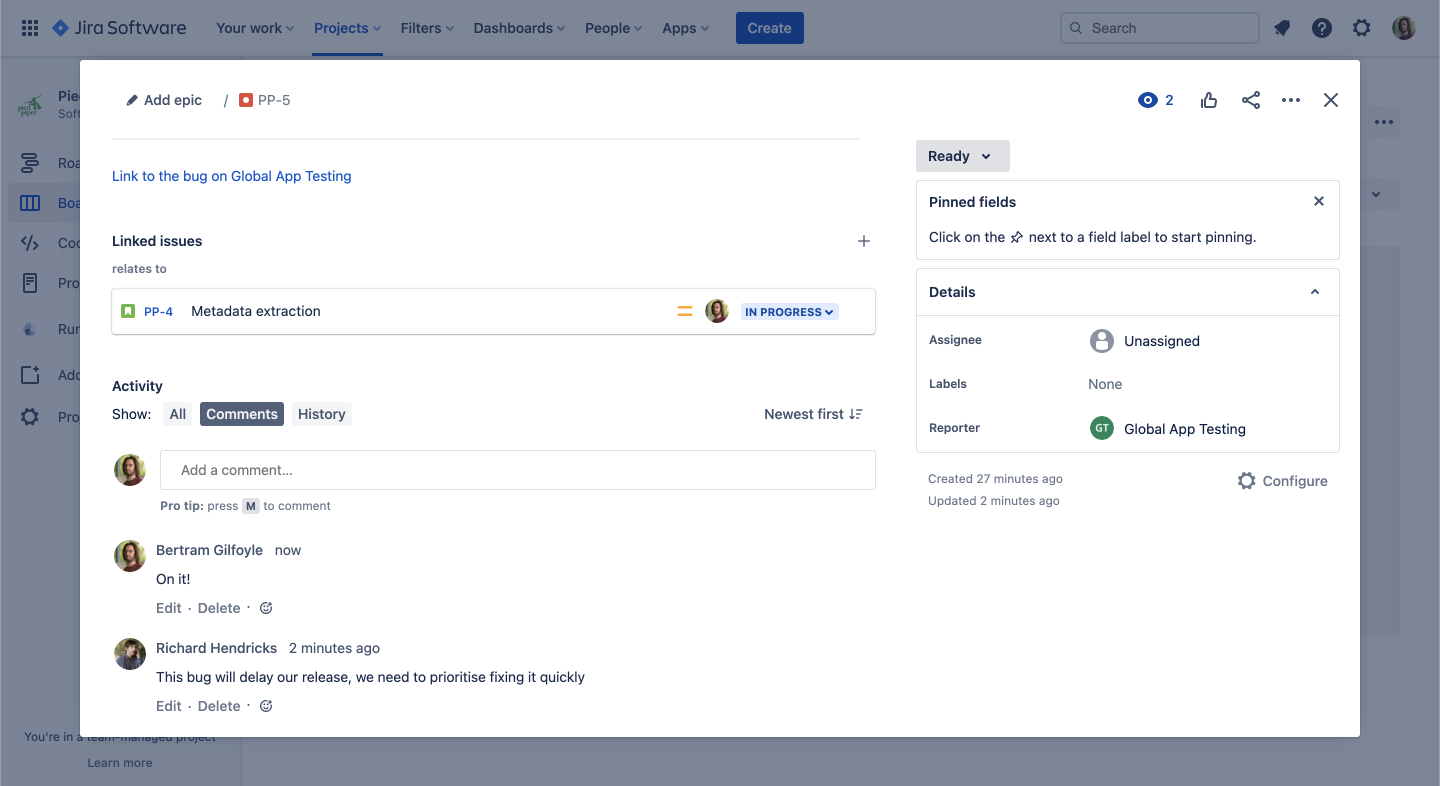This image displays a screenshot of a web page with a pop-up window in the center, captured in a landscape orientation that is wider than it is tall. The background of the web page is slightly grayed out and not in full focus, while the foreground features a detailed interface design.

At the top of the web page, there is a navigation bar that starts with a 3x3 dot grid icon, followed by a blue diamond logo with white text inside. To the left of the logo, it reads "Jira Software." The navigation options available include: Your Work, Projects, Filters, Dashboards, People, and Apps. The "Projects" tab is highlighted with a blue underline, indicating it is currently selected. On the right side of this navigation bar, there is a prominent blue button labeled "Create" in white font.

In the center of the page, dominating the view, is a large, rectangular, white pop-up box. At the top of this pop-up, there's a black "Edit" button and the text "Add Epic." Below it, there is a red box with white text reading "PP-5." Adjacent to this, an eye icon accompanied by the number "2" in blue, a thumbs-up icon, and a share button are visible.

Further down, on the left side of the pop-up, it says "Link to the bug on Global App Testing." A subheader labeled "Linked Issues" follows, with a white box containing black text information. To the right of this box, there's an avatar of a user alongside a blue box indicating the status "In Progress."

At the bottom of the pop-up, there's an "Activity" section with a "Show" dropdown menu and options for "All," "Comments," and "History," with "Comments" currently selected in a black rectangular box with white text. This section shows a series of comments made by various individuals, each accompanied by respective user icons.